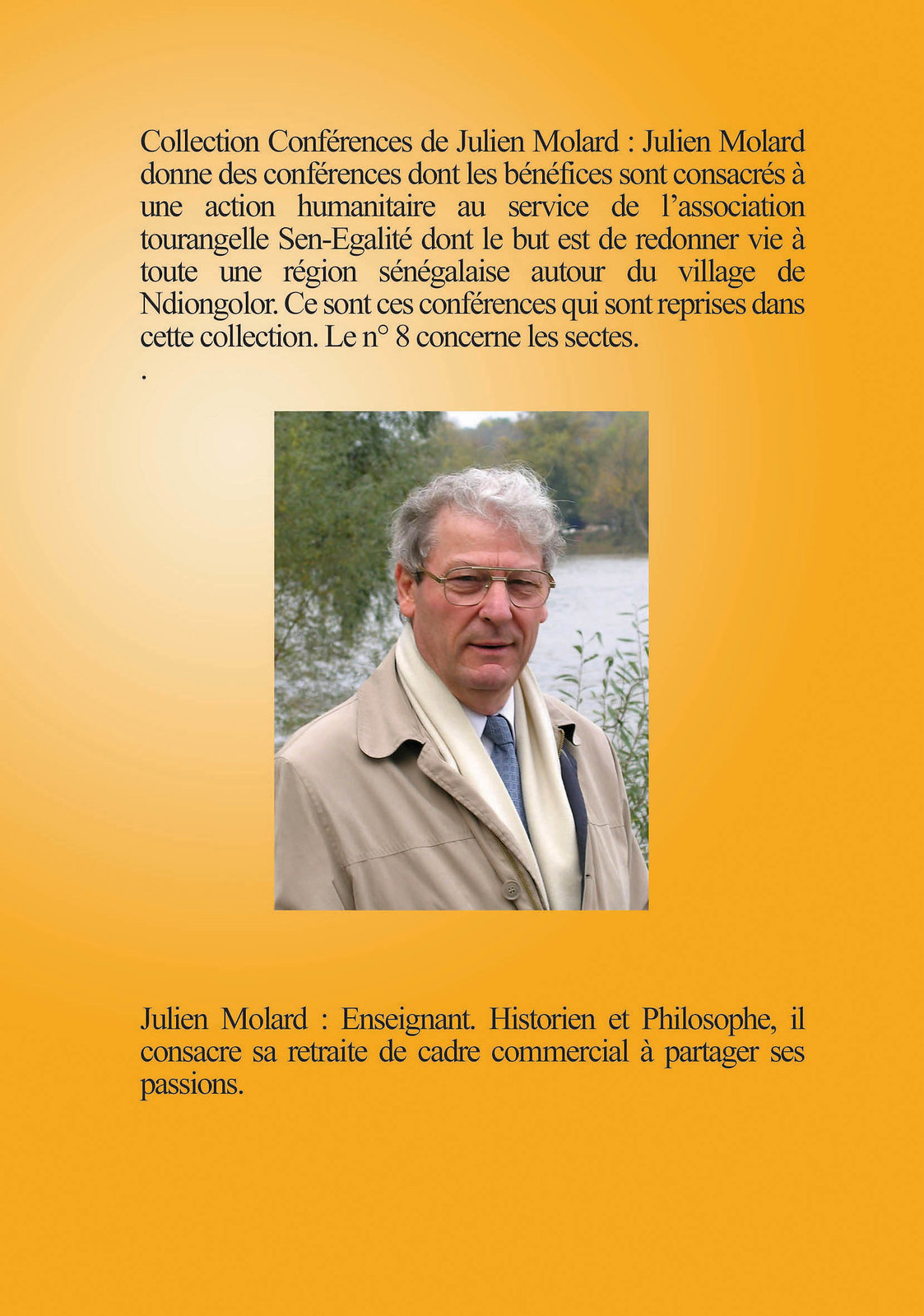This image features a page with a vibrant orange gradient background transitioning from lighter white-orange at the top left corner to a deeper orange on the right. At the top and bottom portions of the page, there are multiple lines of text in French. Centered within the frame is a photograph of an older gentleman, likely in his mid to late 60s, identified as Julian Millard (or Molard). Above the photograph is a paragraph that presumably delves into his biography or achievements, while a smaller paragraph below reiterates his name alongside descriptors such as historian, philosophy, commercial cadre, and passions.

The man stands in front of a picturesque lake with a backdrop of a weeping willow and other trees. He is dressed in a tan trench coat with brown buttons, an ivory-colored scarf neatly around his neck, and a white collared shirt complemented by a blue tie. His appearance is completed with gray, somewhat wavy hair above his ears and silver-rimmed reading glasses. The overall composition and text suggest this might be an obituary or a commemorative page.